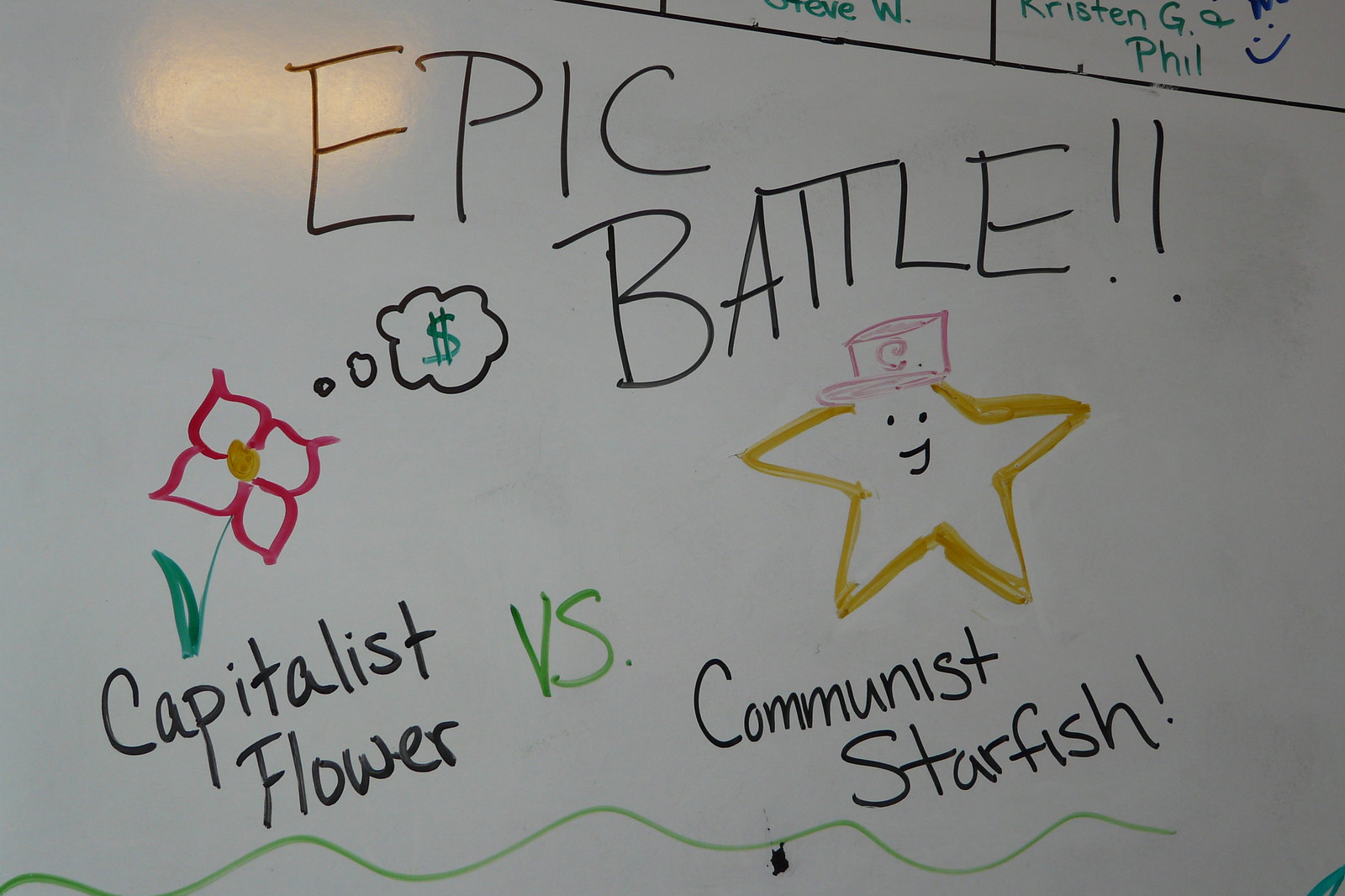The photograph captures a somewhat dirty whiteboard with shaded areas due to lack of light. In the top left corner, a shiny yellow spot reflects light. The top right corner features the bottom of a chart bordered in black with some green marker text and a blue smiley face. Most strikingly, across the top in large, hand-drawn black capital letters, it reads "EPIC BATTLE!!" Just below this, on the left side, is an illustration of a flower with a green stem, red petals, and an orange center, accompanied by a thought bubble with a green dollar sign. Beneath this flower, it says "CAPITALIST FLOWER" in black text. To the right of the flower is the word "V.S." in green text, leading to a depiction of a gold star with a smiley face, eyes drawn as black dots, wearing a red hat marked with a 'C.' Underneath the star, the text reads "COMMUNIST STARFISH!" with an exclamation point. A green squiggly line runs horizontally across the bottom of the whiteboard, tying the composition together.